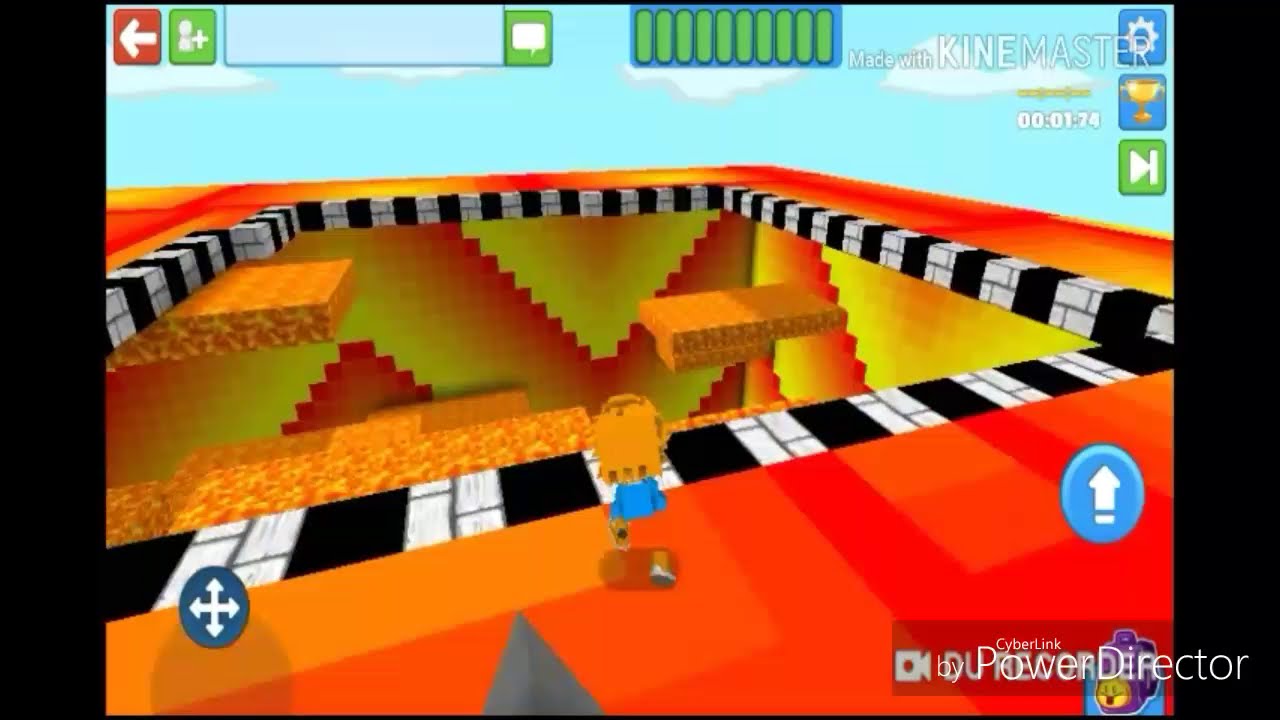This image depicts a simplistic, Minecraft-like video game screen with primitive graphics. The scene features a blue sky with white clouds occupying the upper fourth of the picture, topped by an array of game icons. These icons include a red square with a white arrow, a green square with a figure resembling a person's head and chest, and various navigation buttons like a left arrow and a plus sign. There's also a health meter in the center, and on the right, icons for settings, a trophy, and a forward/fast forward button, each with a blue background. The screen is bordered by thick black lines on the left and right sides.

Prominently displayed at the top right is the text "Made with KineMaster," while the bottom right corner features "CyberLink PowerDirector." The main game scene is a square pit outlined in black and white checkered tiles, giving way to what resembles lava below. Within this pit, there are orange and red-yellow horizontal platforms, some seemingly floating in midair. The design also includes a triangular pattern inside the pit with alternating orange and yellow outlines. Dominating the lower section of the image, a character in a blue shirt with blonde hair stands on an orange floor, with footwear visible against the vibrant background. 

Additional details include the numerical display "00:01:70" near the top and navigation icons in the bottom left corner, emphasizing the game's interface elements.